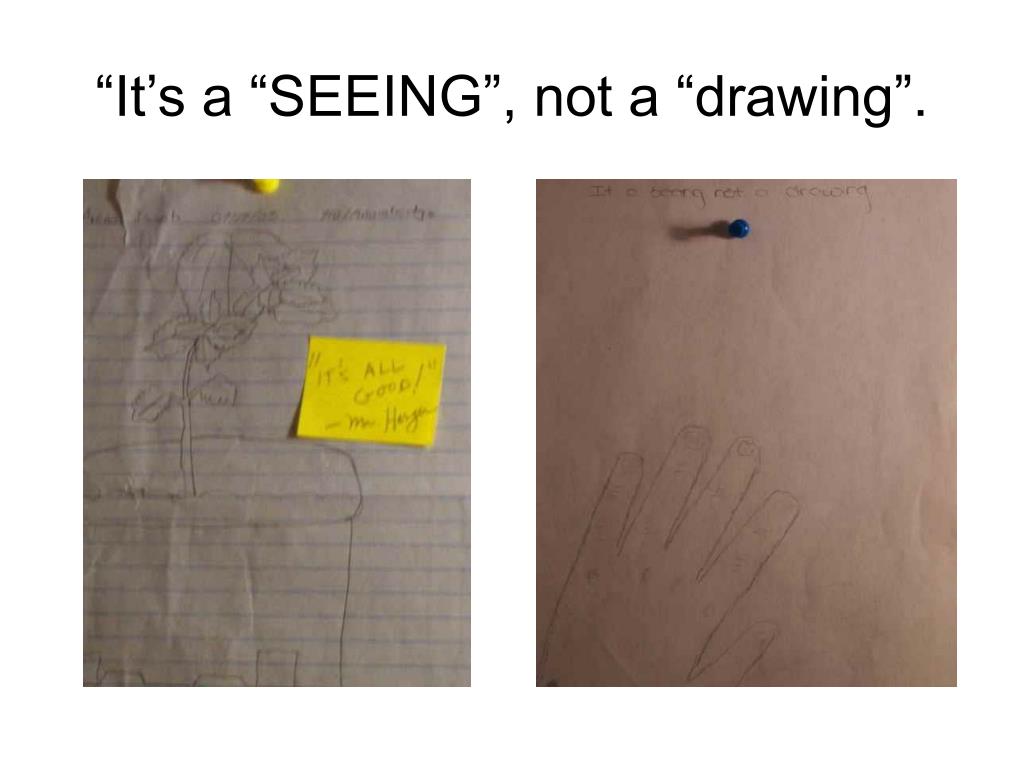The image consists of a composite of two distinct photographs placed side by side, separated by a thick white line, and topped with a white header. The header features black text reading, "It's seeing, not a drawing." The photograph on the left showcases a piece of crumpled and torn notebook paper, pinned by a yellow pin at the top center. The notebook paper contains a pencil sketch of a pot with a flower and multiple buds. Despite the presence of some handwriting at the top, it is too blurry and wrinkled to decipher. Additionally, adhered to the notebook paper is a yellow note that reads, "It's all good." The right photograph displays a clean, white piece of paper with the outline of a hand. Both pieces of paper appear clipped to an unseen surface. The overall arrangement, with its varied colors of black, yellow, and the off-white, suggests the style of a social media post, visually presenting the concept that the hand outline signifies a way of "seeing" rather than just drawing, perhaps hinting at the perspective of a blind person.